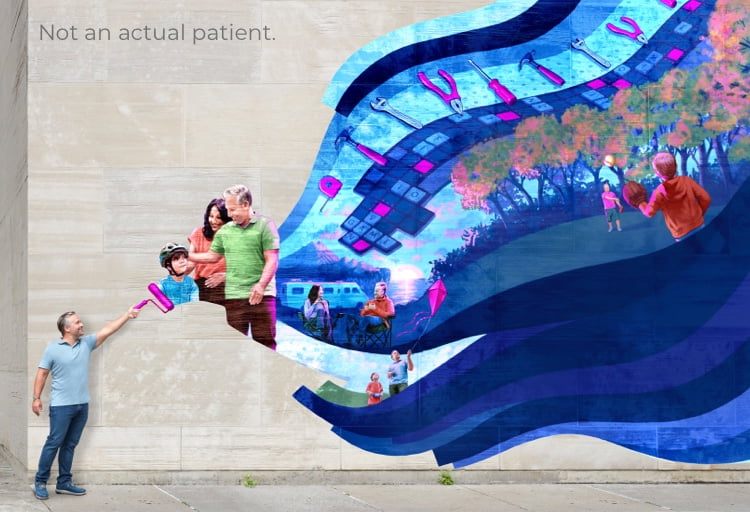The image depicts a digitally crafted mural intended to look like it's painted on the beige cement side of a building with a brownish-grayish block exterior. The mural features a Caucasian middle-aged man in a teal polo, blue jeans, and blue tennis shoes, standing on a sidewalk. He holds a bright magenta pink paint roller in his left hand, extended upward as if painting the mural. The mural showcases a lifelike image of the man in different attire—a green shirt and brown pants—interacting with various family members and scenes that appear to be snippets from his life.

Above him on the mural, there are depictions of a woman with dark hair in a salmon-colored shirt, a little boy in a biker's helmet, and an older lady in a green shirt. They are engaged in activities such as camping, flying a kite, and playing baseball, against waves of blue and hot pink hues. Tools and a Scrabble board are also illustrated, suggesting the man's hobbies and interests. The caption "not an actual patient" is inscribed in the top left corner of the image, hinting at a personal or fictional narrative woven into this vibrant and complex mural.